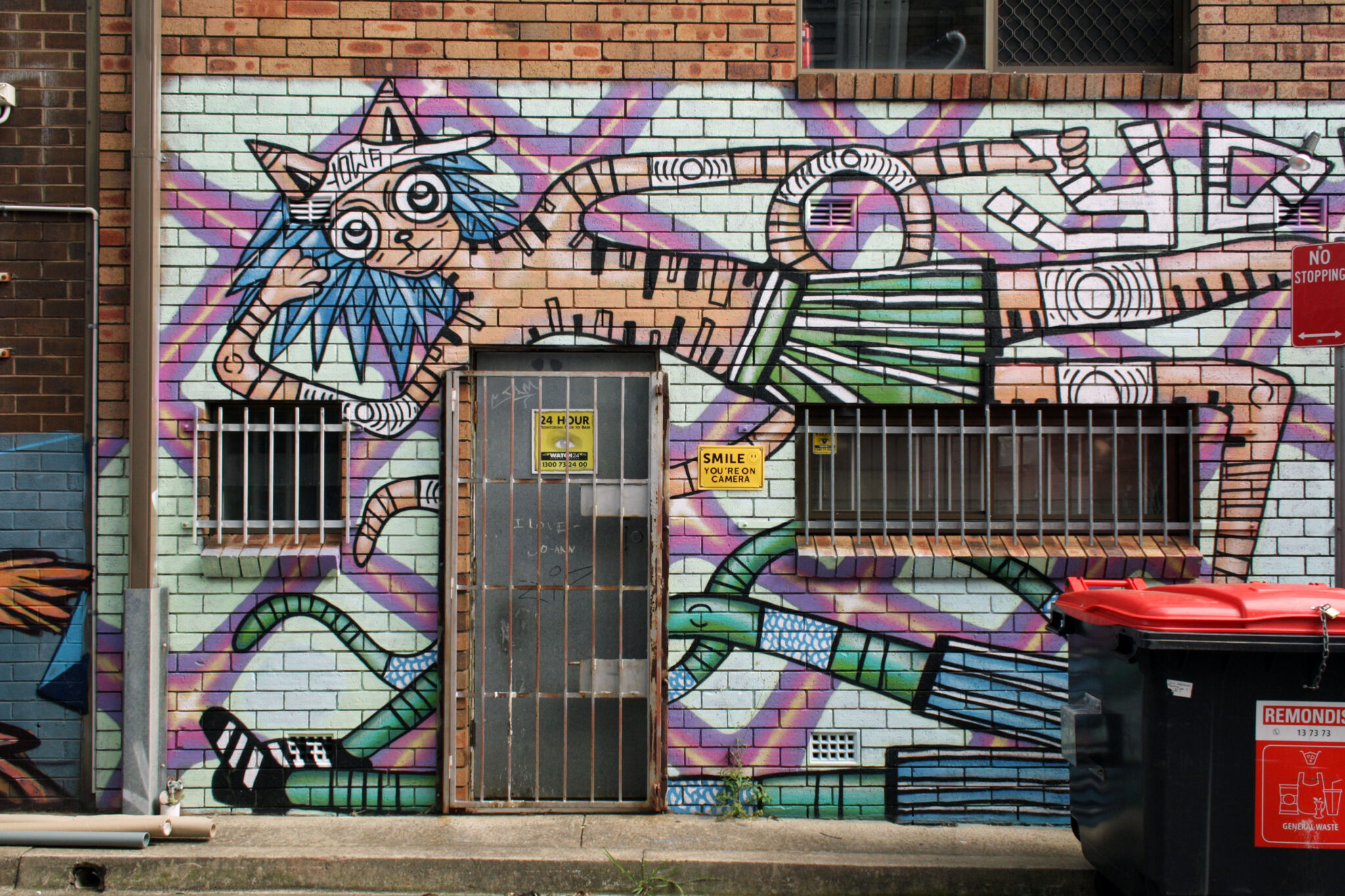In this vibrant photo, the side of a red brick building is transformed by an extensive and artistically vibrant graffiti mural, depicting two cat-faced humanoids. The focal point is an orange, tiger-striped cat figure lounging horizontally with its head to the left and legs to the right, wearing a green and white skirt, knee pads, and a visor hat emblazoned with "Iowa" through which its ears poke. This main figure grips a stylized white letter "Y" in its right hand, with an adjacent letter "O." Another green, tiger-striped cat figure appears from ground level, though it is partially obscured by a black and red garbage bin in the foreground. Barred windows of differing heights flank a central barred doorway, adding to the urban, city environment. The entire scene is set against a white background crisscrossed with dynamic purples, pinks, and gold geometrical shapes, giving a cartoonish, animated essence to the otherwise industrial setting.